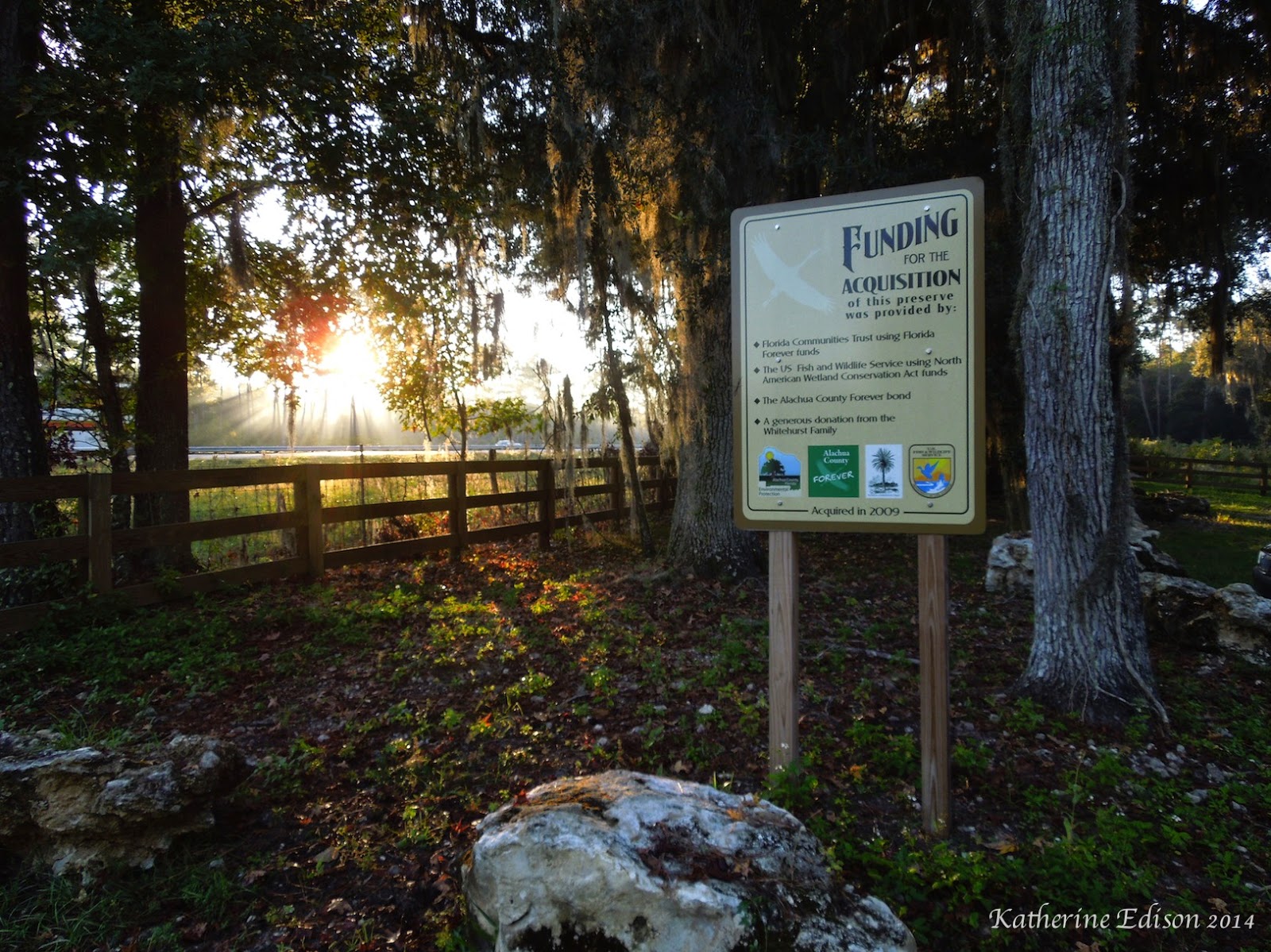In this detailed outdoor scene, a sign mounted on two wooden posts stands near the middle right-hand side of the image. The sign reads, "Funding for the acquisition of this preserve was provided by," followed by four bullet points beneath blue lines, detailing contributors. Below the text, there are four images: one depicting a person, a second with a green background, a third featuring a tree, and a fourth, patch-shaped, possibly depicting a bird. The bottom of the sign indicates the preserve was acquired in 2009. In the lower right-hand corner, "Catherine Edison 2014" is inscribed in white text.

The foreground is dominated by a large white rock on the left side, surrounded by an area dense with grasses, weeds, and other vegetation. Toward the middle of the frame stands a wooden fence with scattered posts and three horizontal boards stretching across it. Tall trees flank the scene: one trunk on the right side is particularly prominent, while in the center, additional tree trunks with hanging branches appear thick and robust. Tree trunks are also visible on the left side, and sunlight filters through the foliage, casting dappled light across the ground.